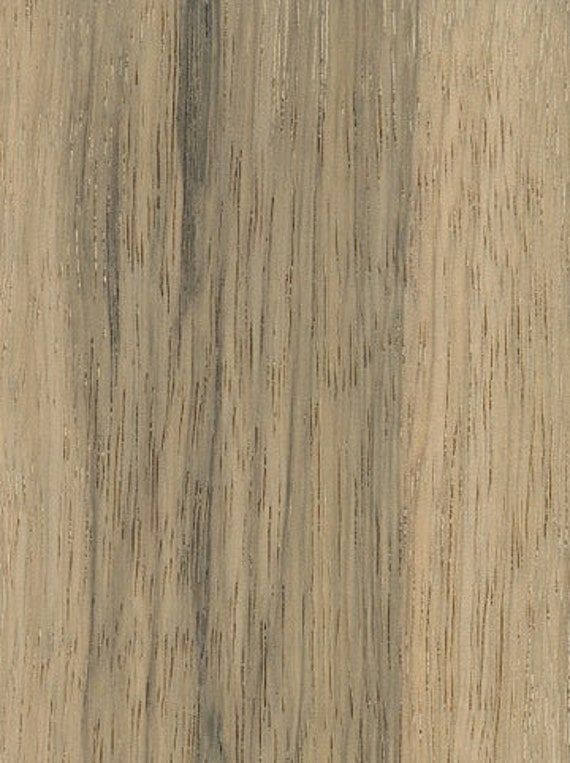This close-up photograph captures an intricately detailed piece of wood or a wood-like surface, zoomed in to the point where the medium—whether it's an actual plank, a photograph, a painting, or a linoleum imitation—is indiscernible. The image reveals a rich tapestry of vertical wood grain, prominently showcased in varying hues. The primary color is a medium beige, transitioning to a darker, gray-charcoal tone with a distinctive greenish tint that dominates the central two-thirds of the frame. This darker hue is interspersed with thin, thread-like strands of dark brown, adding to the complexity of the grain. The lighter beige is more pronounced on the right and left edges, with the center showcasing the deeper, variegated colors. The stippling, or textured grain of the wood, is vividly apparent, giving the surface a non-uniform yet harmonized appearance that ranges from blonde to dark beige-gray. Each detail, from the fine brown lines to the subtle greenish undertone, provides a striking visual that emphasizes the wood’s natural, intricate beauty.